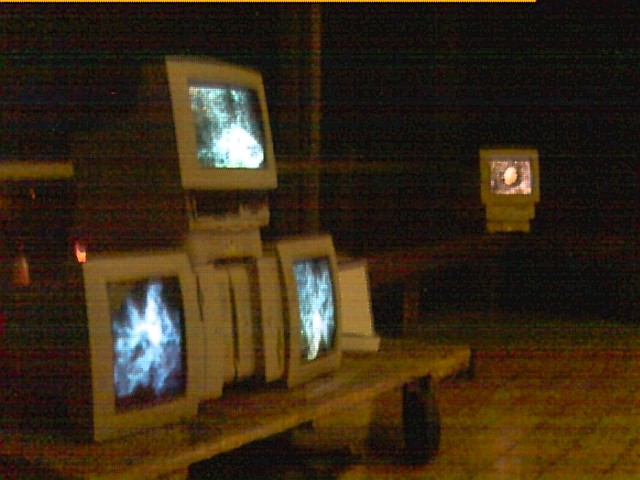The image depicts a nostalgic scene with a sepia-toned composition, featuring a set of three old CRT monitors stacked in a pyramid-like arrangement on a thick, low table with tiled flooring visible. The two monitors at the base lie sideways, facing outward, while the one on top stands vertically. These monitors display unclear black-and-white images, possibly medical scans or internal structures. The photograph gives an impression of being an old, degraded color print with streaky lines, suggestive of low resolution or damaged quality akin to early 1990s video screenshots. Additionally, another CRT monitor is seen distantly, positioned on a separate shelf, facing the viewer with a bright object on the screen against a darker background, potentially resembling a face, fruit, or ball.